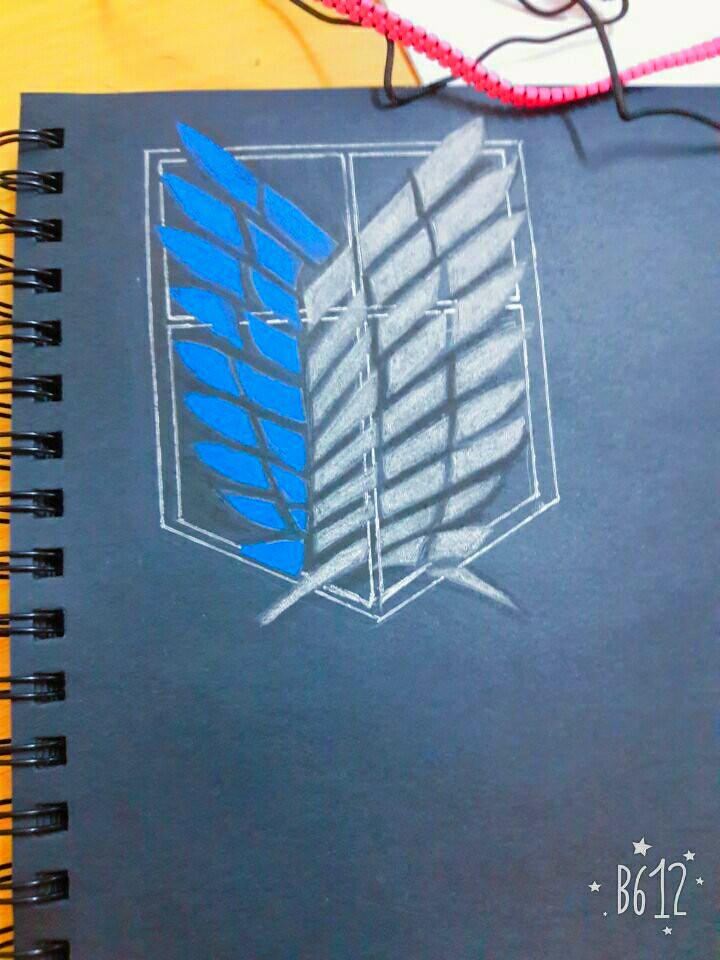Photograph of a dark navy-blue spiral notebook with visible black metal spirals along the left side. The notebook's cover features a detailed drawing outlined in white, resembling a house structure: a square top with a pointed bottom, containing four pane-shaped sections. Each section has intricate blue and white feather-like designs, with the blue feathers on the left and the white ones on the right. The bottom right corner displays the text "B612" surrounded by small white stars. The background features a mustard yellow color on the left side, transitioning to white on the right, with a thick pink spiral cable at the top and thin black pieces scattered around.